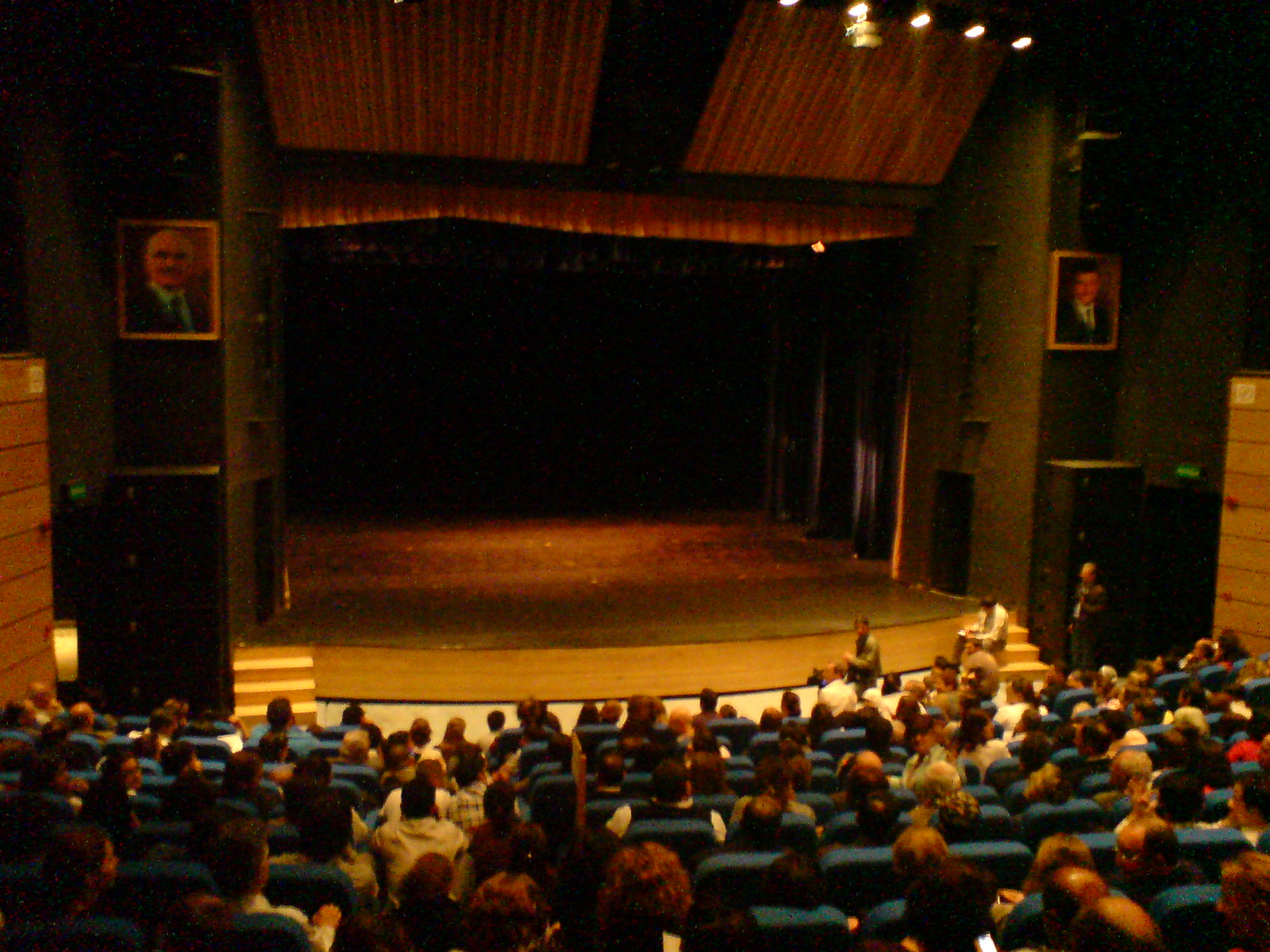The image depicts an auditorium with a stage set against a deep, dark backdrop and framed by brown curtains. The stage, which appears approximately 20 feet deep, features a polished hardwood floor and is flanked by pairs of stairs on either side, each with three steps. On the stage's left and right sides, there are framed portraits of men in suits, possibly depicting important figures or related to the theater. 

From a mid-back, elevated audience perspective, we can see rows of blue cushioned chairs, about 65-70% of which are occupied by people, who appear to be awaiting the start of an event. There's a noticeable gathering of audience members, and several individuals are positioned near the stage, including a man in a white shirt and tan pants seated on the right side stairs and another person standing behind him, possibly a stagehand or producer. The overall atmosphere suggests anticipation of an upcoming performance with accent lighting highlighting the stage.